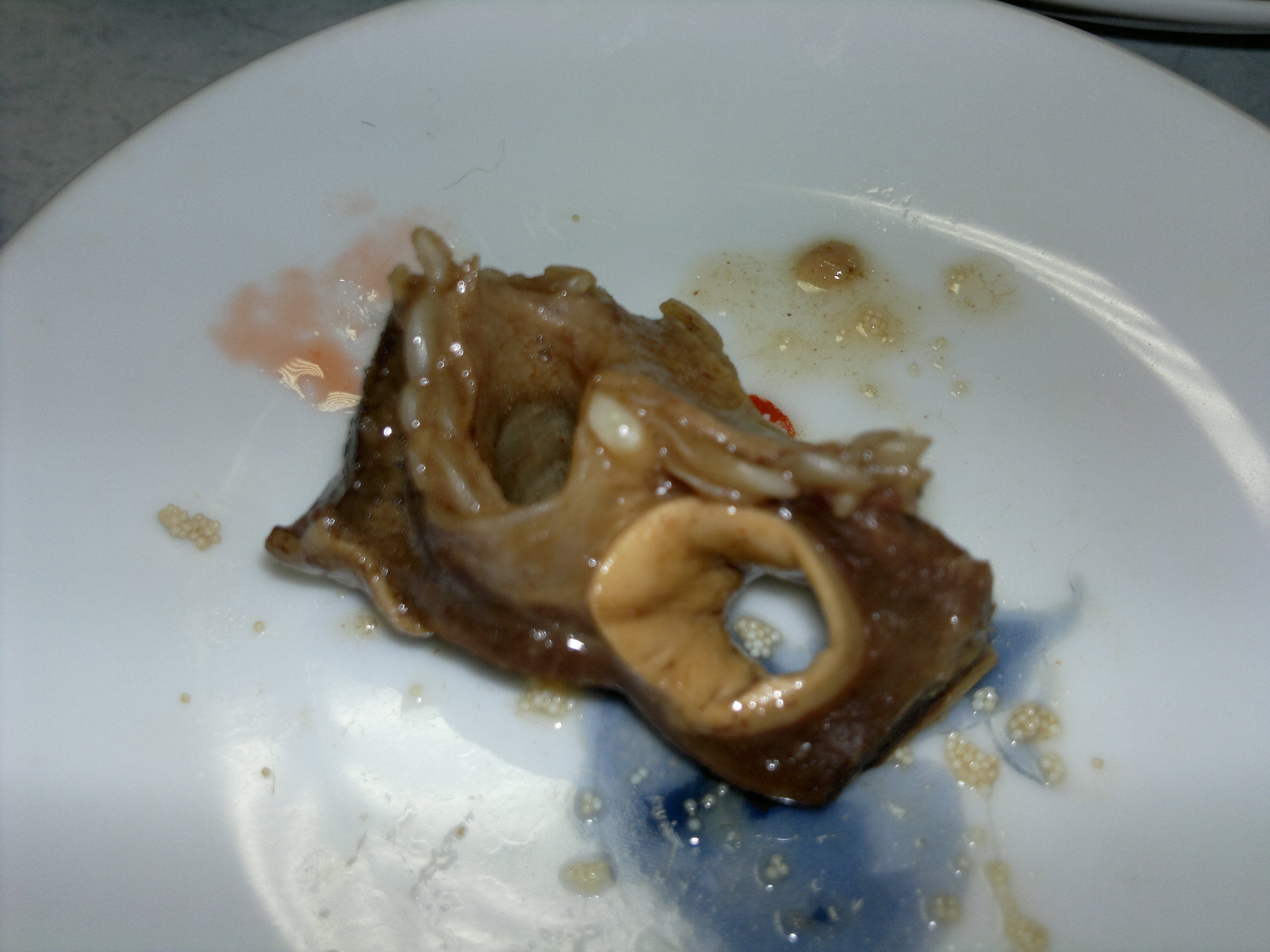In this detailed photograph, we see a white plate resting on a gray surface, possibly a table or counter. On the plate lies a peculiar piece of food, which appears to be some kind of meat, perhaps resembling an intestine or a piece of cooked steak with varying shades of dark brown and white tinge. The meat is adorned with what looks like blue and pink sauces drizzled over its surface, adding a confusing element to its appearance. Scattered around it are tiny white specks, which could be caviar or fish eggs. There are distinct features such as possible suction cups and a hole, suggesting that it might be a part of an animal, like an octopus. On closer inspection, the upper left-hand side of the meat shows what appears to be teeth. The plate looks somewhat messy with crumbs and grease, indicating that most of the meal has already been eaten, leaving behind this unappetizing piece of food.